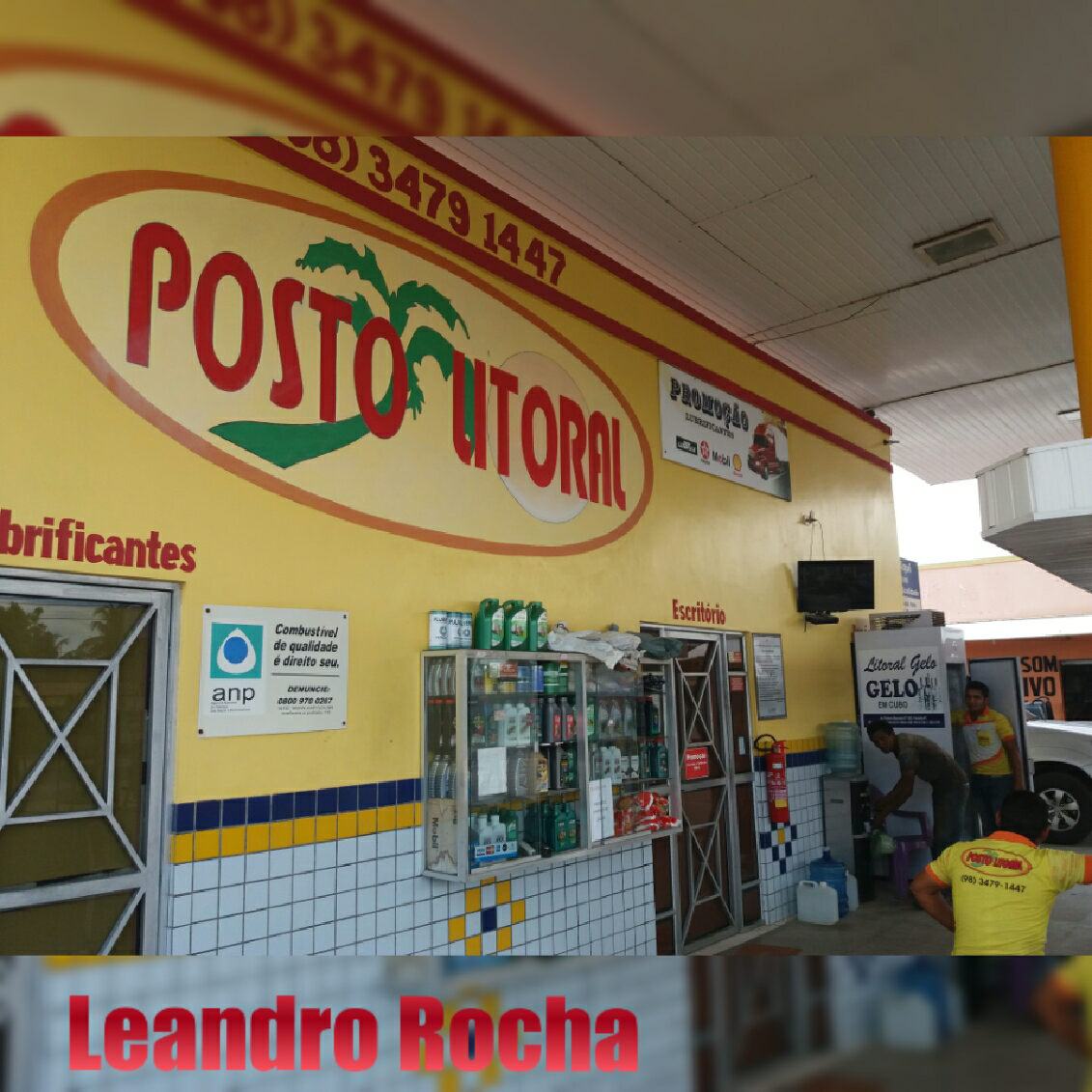This image depicts the exterior of an automotive service store named Posto Littoral, as indicated by the prominent logo featuring a bent palm tree and the words "Posto Littoral." Above the logo is the phone number 3479-1447. The store's facade is predominantly yellow, with a section at the bottom adorned with blue, white, and yellow tiles. Several shelves mounted on the wall hold various engine oils and other automotive liquids. A fire extinguisher is affixed to the wall near the main entry door, which is currently closed. In front of the store, a few people are engaged in their tasks, with two individuals wearing uniforms displaying the same store logo. Additionally, a vehicle can be seen in the background, likely being serviced. The bottom left corner of the image bears the red text "Leandro Rocha." This comprehensive scene captures a busy moment outside the store, highlighting its automotive-oriented services and vibrant exterior.